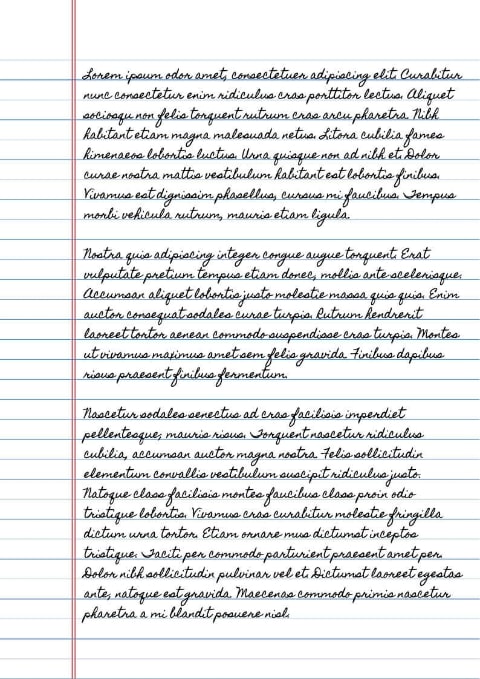The image is a color illustration of a piece of college-ruled paper against a plain white background, measuring approximately five inches high by four inches wide. The paper features alternating light blue and slightly darker blue horizontal lines. On the left-hand side, about three-quarters of an inch from the edge, there are two thin vertical red pinstripe lines that extend slightly above the topmost horizontal line and meet the bottommost line. The paper contains three paragraphs of small black cursive writing, starting on the second line from the top and situated to the right of the red lines. The text is in a foreign script, rendering it illegible and suggesting it might be "Lorem Ipsum" filler text. This handwritten font exhibits variations in individual letters, indicating it as a designed template, possibly for graphic design or notebook product photography. The final paragraph ends three lines before the bottom of the page, further emphasizing the detailed, floating appearance of the paper against the white backdrop.